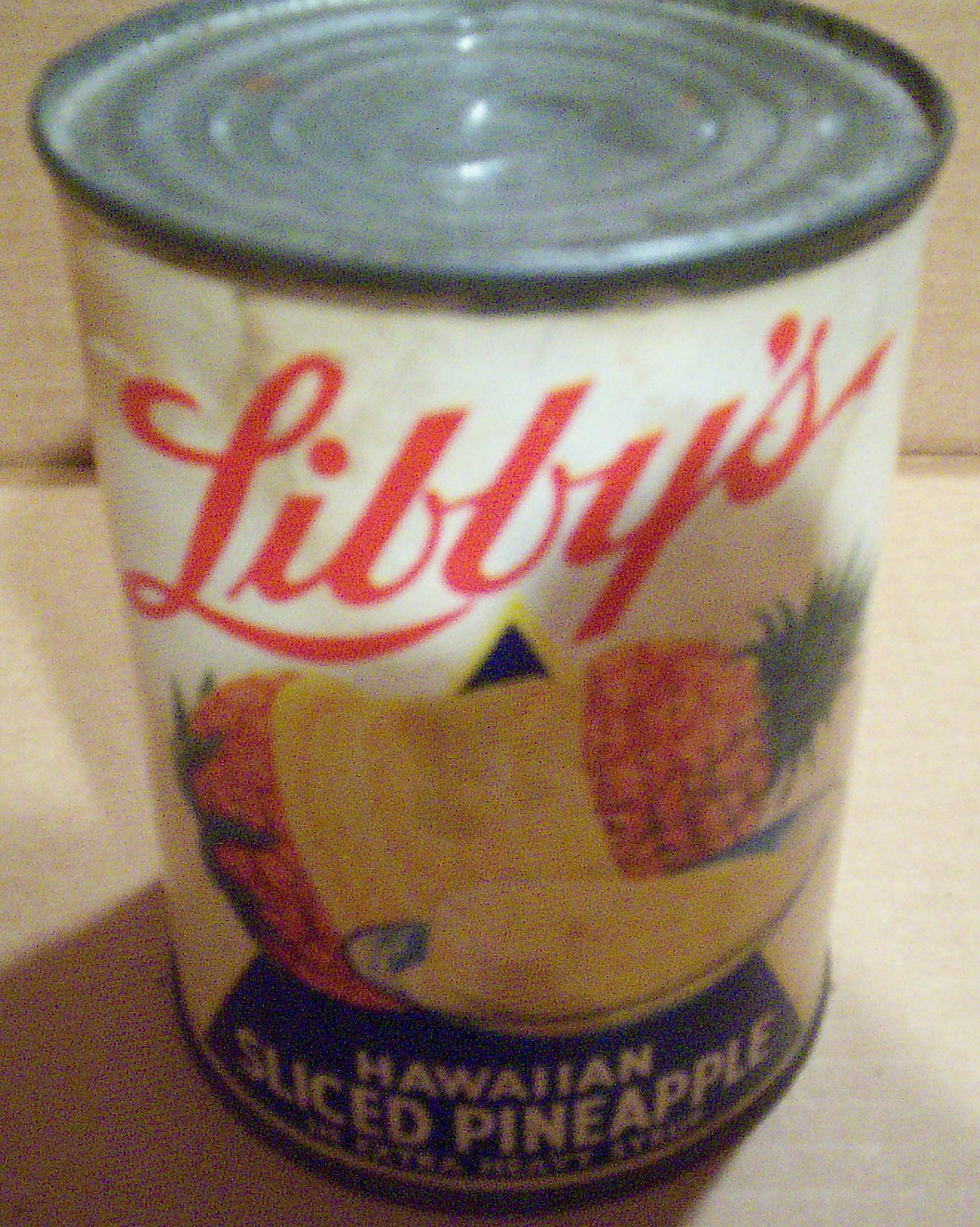The image features a close-up of a vintage can of Libby's Hawaiian Sliced Pineapple, situated on a white countertop with a tan background. The can itself exhibits signs of aging, with a darker gray lid speckled with rust-like spots and a slightly wrinkled label. The label, viewed from a slightly downward angle, predominantly features a white backdrop. A blue triangle at the bottom of the label displays the text "Hawaiian Sliced Pineapple" in bold white block letters, along with a note indicating the presence of "extra heavy syrup." Above this text is an illustration of a whole pineapple, positioned sideways with its leaves pointing to the right. This pineapple is depicted in a tannish-orange hue, with a prominent sliced chunk of the juicy yellow fruit prominently displayed. The brand name “Libby's” appears in elegant red cursive lettering, prominently positioned above the pineapple illustration.